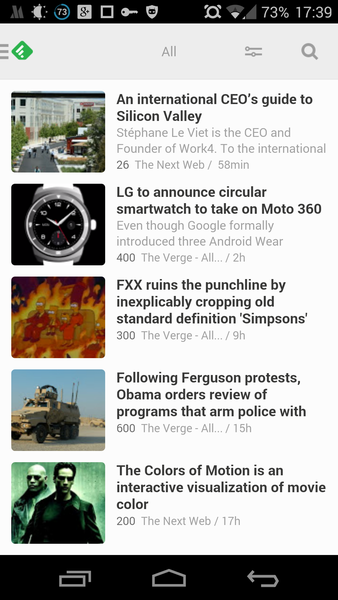The image depicts a smartphone screen displaying a variety of notifications and content. 

At the very top, a black banner spans the width of the screen, filled with various icons. These include Google, a moon symbol (likely indicating a Do Not Disturb mode), an alarm clock, Wi-Fi signal strength, network connection strength, and battery status. The time is displayed on the far right as 17:39, next to a battery indicator showing 73% remaining.

Below the black banner is a light grey panel featuring a few options, including a prominent search bar.

The main content area under the grey panel is filled with a series of stories, each represented by a tiny picture on the left followed by a headline and a brief descriptive text. 

1. The first story displays an image of a street scene with the headline "An International CEO's Guide to Silicon Valley."
   
2. The second story features a picture of a watch, with the heading "LG to Announce Circular Smartwatch to Take on Moto 360."

3. The third story appears to be a scene from "The Simpsons," with the headline "FXX Ruins the Punchline by Inexplicably Cropping Old Standard Definition Simpsons."

4. The fourth story shows an image of an armed truck, bearing the headline "Following Ferguson Protests, Obama Orders Review of Programs That Arm Police."

5. The final story features an iconic scene from The Matrix movie, with the heading "The Colors of Motion is an Interactive Visualization of Movie Color."

The stories layout reflects the diverse and topical nature of the smartphone user's interests and trending news items.